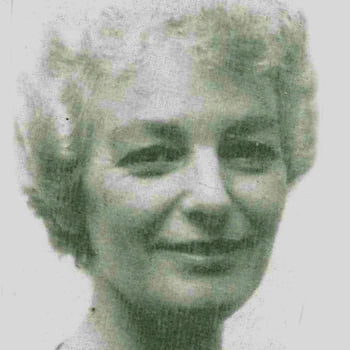This is a black and white photograph of a woman, captured from slightly below the chin to just above the top of her head, which is partially cropped out. The image, which has an off-white, plain background, is somewhat grainy and shows signs of wear and tear with heavy shadowing and a faded hue. The woman has short, wavy or curly hair that falls just below her ears and down to the back of her neck. Her hair appears light-colored, possibly blonde or gray. She is smiling warmly, showing a couple of her front teeth. Her head is turned toward the camera, but her body is slightly angled, creating a soft, engaging posture. There is also a mole visible on the right side of her neck. Overall, she exudes a sense of happiness despite the picture's age and condition.